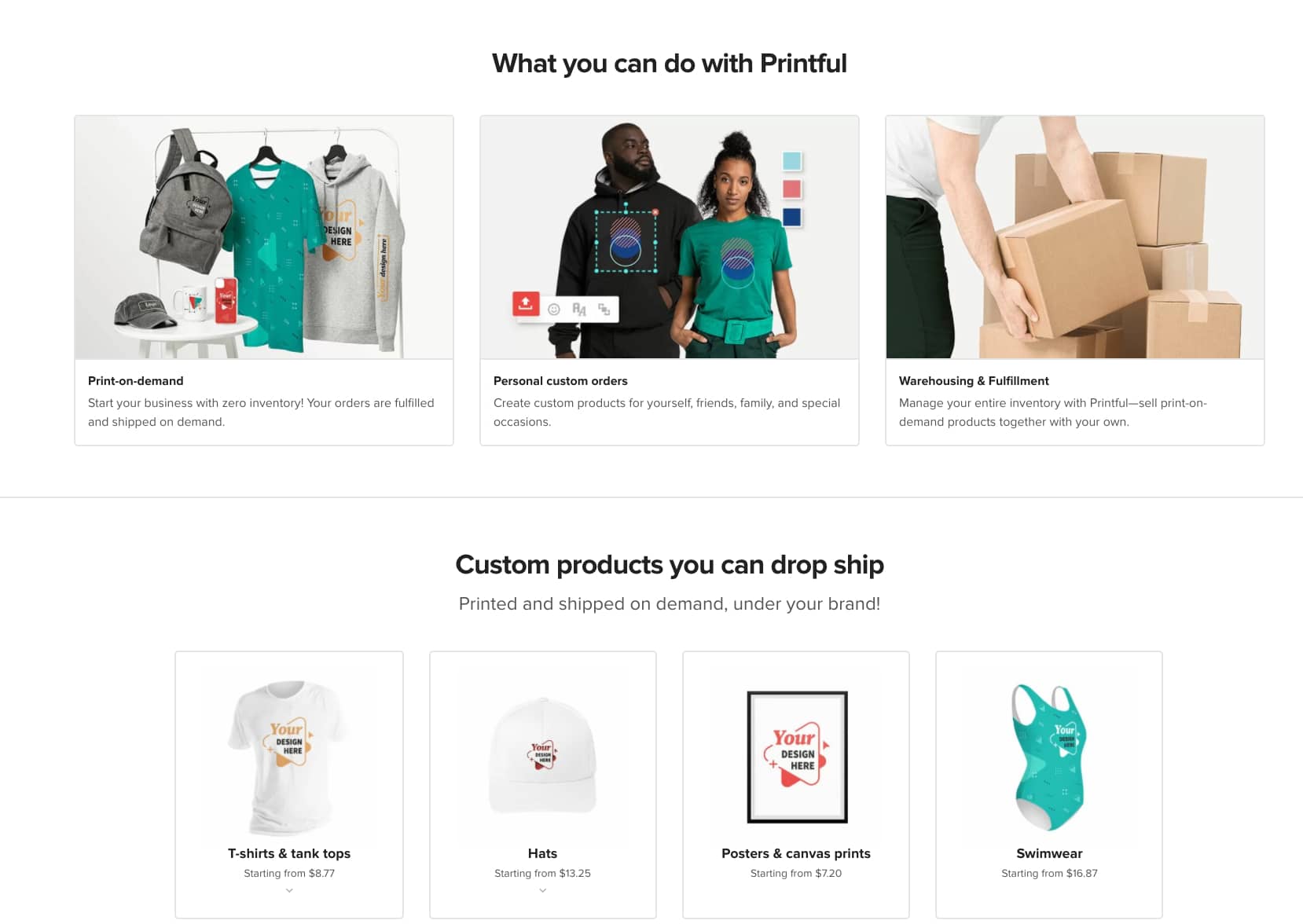Discover the possibilities with Printful's Print on Demand services—ideal for starting your business with zero inventory. The image showcases a vibrant green t-shirt with a circular design print, featuring hands casually placed in the pockets. The t-shirt is adorned with blue and red accents. 

Printful allows you to fulfill and ship orders on demand, perfect for both personal and custom orders. You can create unique products for yourself, friends, family, and special occasions. The service also includes warehousing and fulfillment, where you can manage your entire inventory with ease. 

Advertised on the shirt are options for custom products, including t-shirts, tank tops, pants, boots, camisoles, and swimwear with prices starting from $3.25 to $16.87. The shirt features a variety of geometrical designs, including squares and circles, which highlight the customization possibilities. The image effectively showcases the versatility of Printful for drop-shipped, print-on-demand products tailored to your brand.